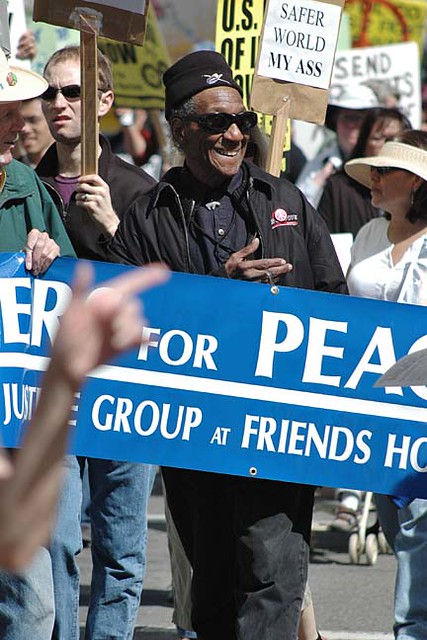The photograph captures a peaceful protest or rally, held outdoors during the day, characterized by a diverse group of participants. Central to the image is an elderly Black man, likely in his 60s, with grayish hair peeking out from under a black fez-like hat. He is wearing dark sunglasses, a black jacket, a dark button-down shirt, and black jeans. He stands out, smiling and looking to his left, while helping to hold a large blue banner with white text partly visible, ending in "ER for PEACE," and a subheading that includes "Justice Group at Friends, H-O." Also holding the banner, on the left side of the frame, is a man in a green shirt, jeans, and a straw or cowboy hat, although he is mostly cut off. Behind them, other participants are visible, some holding signs affixed to wooden sticks. One prominent sign reads, "Safer World My Ass." The overall scene is calm and underscored by varied colors including shades of blue, gray, green, tan, and black, suggesting a vibrant and engaged crowd.